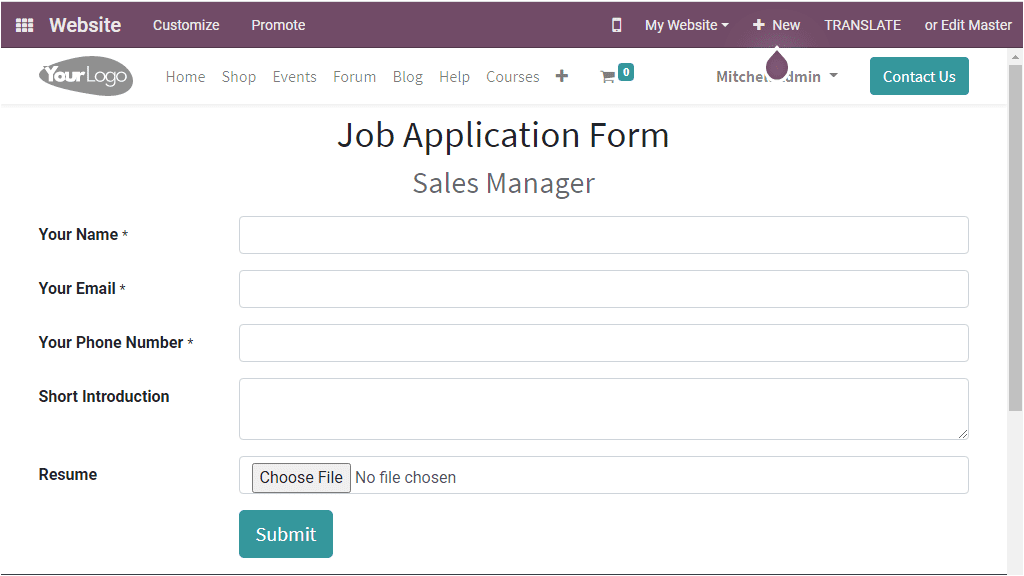This is a detailed screenshot of a job application form for a Sales Manager position on a website. The image is rectangular and prominently features a purple color scheme, a white background, and blue buttons. At the very top of the page is a navigation bar labeled “Website,” “Customize,” and “Promote.” To the right of this bar is a phone icon, and next to it is a drop-down list labeled “My Website.” 

Additionally, there is a plus sign for adding new items, a Translate button, and an Edit Master button. Directly below the Edit Master button is a blue button labeled "Contact Us." On the left side, part of a name, presumably "Mitchin Admin," is visible. 

Beneath the purple navigation bar is an area designated for uploading a logo, indicated by the prompt "Submit your logo." The main website menu includes tabs for Home, Shop, Events, Forum, Blog, Help, and Courses.

The primary focus of the screenshot is the job application form for the Sales Manager position, located under this menu. The form allows users to input their name, email, and phone number, as well as provide a short personal introduction. There is also an option to upload a resume. Completing the form involves clicking a blue “Submit” button located at the bottom.